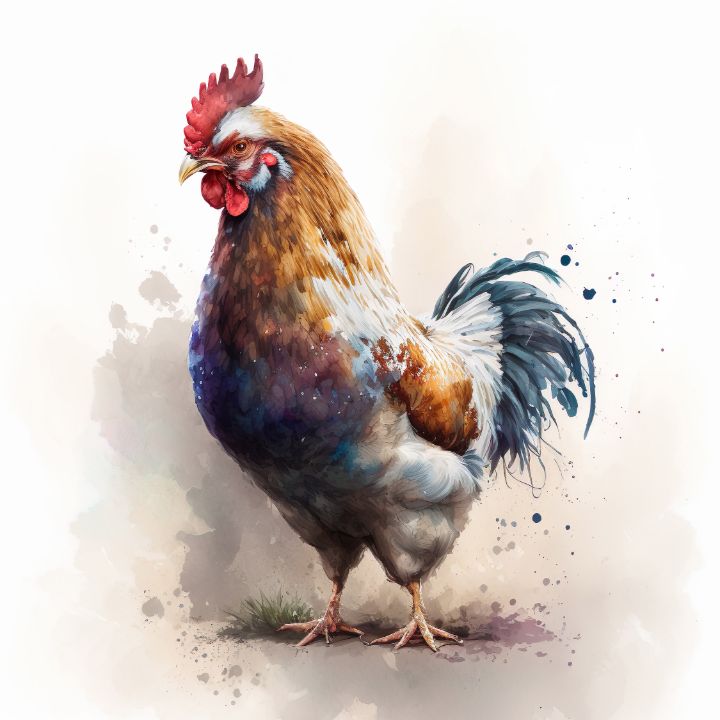This vibrant painting depicts a colorful chicken—possibly a rooster—standing amid splashes of grass and dirt on a textured background. The chicken showcases an array of exaggerated yet stunning colors: its body is predominantly a blend of brown, white, and hints of purplish-brown, while its tail feathers are a mix of bluish-gray and white. The face features striking brown and white patterns with a brown mask, accentuated by a bright red comb and wattles hanging beneath a yellow beak. The background transitions from a white at the top to a dusty cream and brown towards the lower parts, adding to the earthy aesthetic. Paint splatters in shades matching the chicken’s plumage are scattered around, enhancing the overall dynamism of the scene. The perspective gives us a frontal view with a slight angle, capturing the chicken’s serene stance as it faces us while slightly turned to its right.